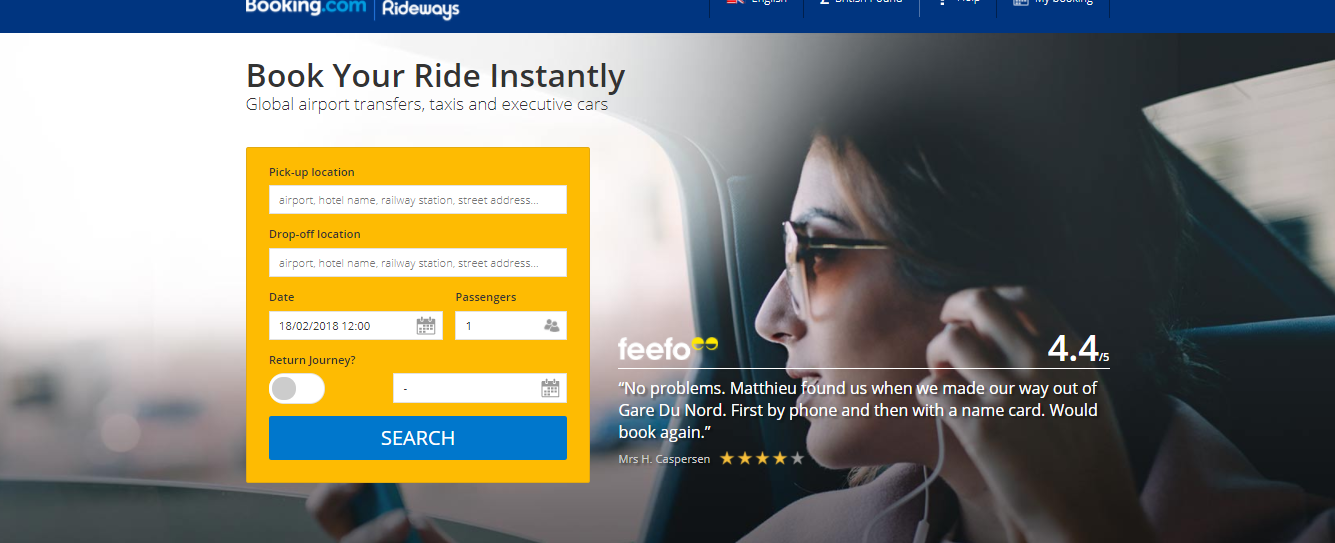This image features a screenshot from the Booking.com website, specifically from the Rideways section. The header includes a partially visible blue bar extending across the top with a portion of icons cut off, yet noticeable by their bottom edges. The identifiable 'Booking.com' logo is also slightly truncated. 

Centered within the screen, prominent black text reads "Book your ride instantly" followed by smaller descriptive text, "Global airport transfers, taxis, and executive cars." Below this, a yellow box requests the "Pick-up location," accompanied by a white input field for users to enter their name and street address. Adjacent to it is a similar section for the "Drop-off location," where users would input their destination details.

Further down, input fields for "Date" and "Passengers" are pre-filled with one passenger, and an option for a "Return journey" can be toggled. Another unfilled white box with a house icon is present, indicating additional information entry.

Beneath these sections is a large, blue search bar alongside an image of a woman sitting in the back of a car, holding a wired earbud to her ear. 

A customer testimonial is displayed below: "Feel foe, no problems. Matthew found us when we made our way out of Gare du Nord, first by phone and then with a name card. Would book again." The feedback concludes with a rating of 4.4 stars.